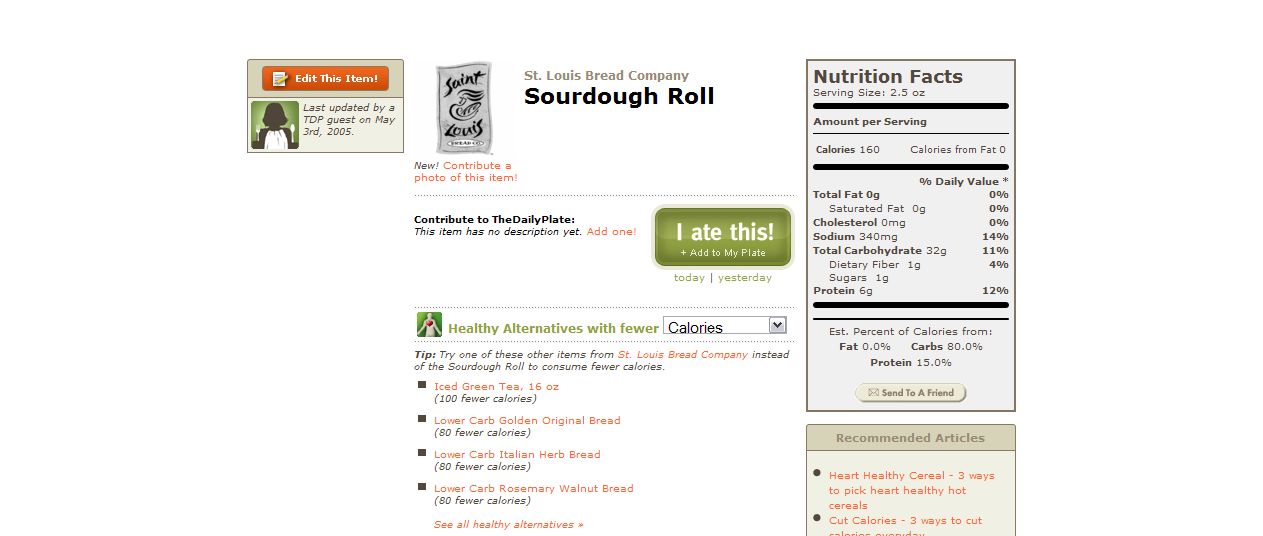The image depicts an online dietary tracking system, possibly from a recommendation website or app. At the center of the interface is a prominent green button labeled "I ate this. Add to my plate," suggesting a method for users to log their food intake. To the left of the button, there is a box featuring an orange and green olive color scheme with an option to "edit this item." On the right side, nutrition facts are displayed, providing detailed information about the food item. Below the nutrition facts, there is a section for recommended articles. At the top of the image, a cartoon design accompanies the text "St. Louis Bread Company Sourdough Roll," identifying the food item featured on the page.